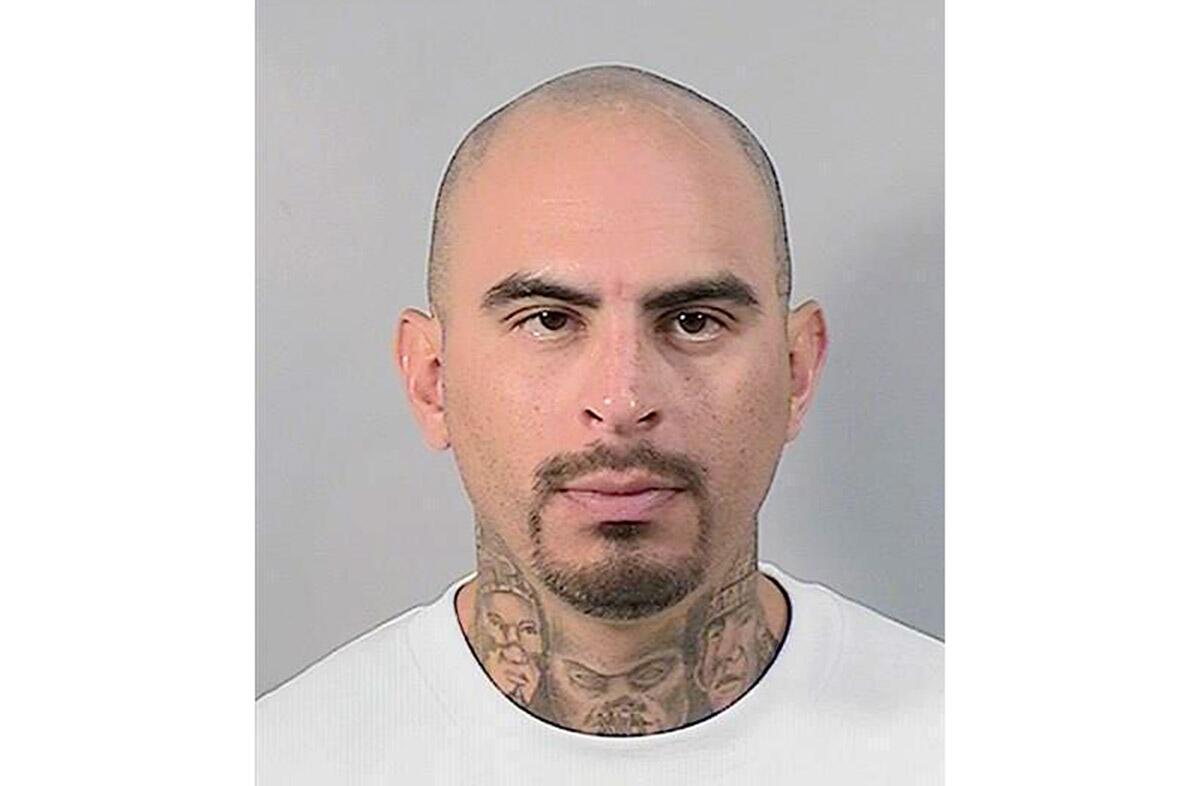The image is a detailed headshot of a white-skinned man, likely a mugshot, against a plain grey backdrop. The photograph captures his head and the top portion of his neck going down towards his shoulders, as seen in passport photos. He has a shaved head with a slight shadow indicating some hair growth, a goatee beard, and a moustache. His left eye, from our perspective, looks upwards towards the ceiling while the right eye stares directly at the camera, suggesting he may have a lazy eye. He is dressed in a white, round-necked jumper. Prominently featured on his neck are tattoos of three distinct faces. The central tattoo depicts a face with lips sewn shut, positioned where his Adam's apple would be, while the other two on either side resemble Native American figures adorned with large hoop earrings, face tattoos or markings, and headdresses. His general facial features, including eyebrows, nose, lips, and ears, appear typical.